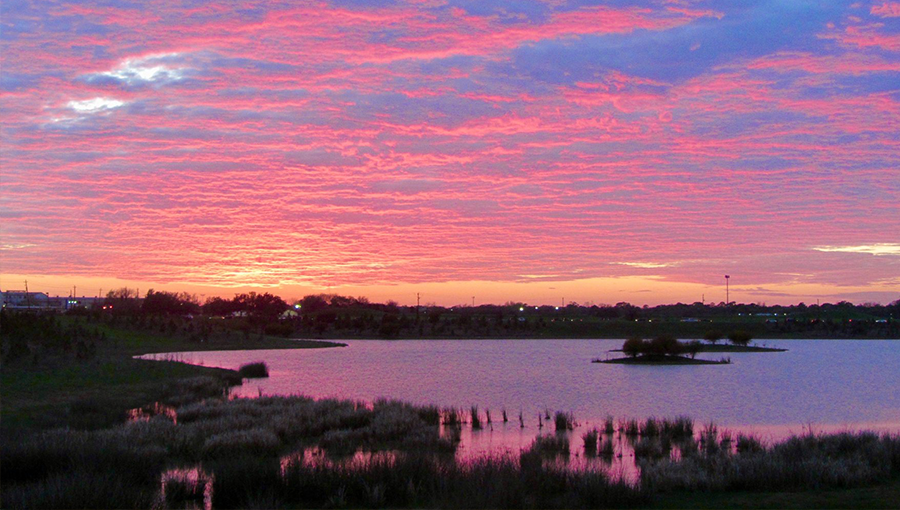A breathtaking sunset illuminates the sky over a modest-sized lake, casting a stunning array of colors that blend seamlessly from pink and orange to hints of purple and blue. The horizon is a vivid stripe of medium orange, marking where the sun has just descended. The sky is adorned with layers of mid-level clouds, each reflecting the sunset's brilliant orange, pink, and yellow hues, creating an almost creamsicle-like complexion across the heavens.

The tranquil lake mirrors this vibrant spectacle, its waters touched with tinges of purplish orange, adding depth and serenity to the scene. Scattered across the water are small islands and patches of grass, suggesting a shallow, marsh-like environment reminiscent of Florida's Everglades. The lush vegetation of green trees and bushes frames the foreground, enhancing the natural beauty of the landscape.

In the distance, the faint outline of a city or possibly a road is visible, with tiny specks of light from radio antennas and streetlights dotting the horizon, providing a subtle juxtaposition between nature and human presence. This landscape-oriented photograph masterfully captures the serene elegance and captivating colors of a sunset over a tranquil lake, making it the focal point of this mesmerizing scene.